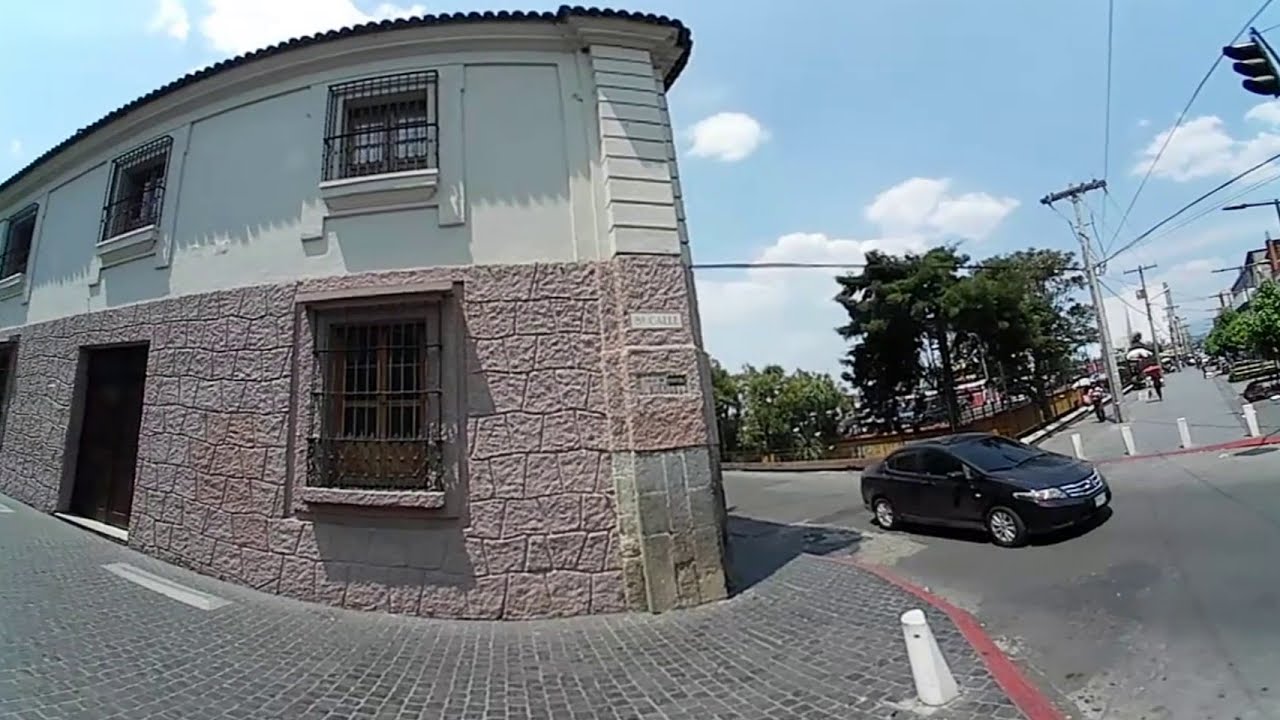This photograph, taken with a fisheye lens, captures a detailed, ground-level view of a curved road bordered by both a sidewalk and a building. The road, painted green, features a black coupe driving to the right. Adjacent to the road, there are several car stopper pillars and scattered pedestrians, including a person with a pink umbrella and another in a white and striped shirt. To the sides of the road stand tall trees and electrical poles with numerous wires extending from them.

On the left side, the focal point is a two-story building. The lower half of the building is constructed from uneven light red bricks, while the upper half is smoothly white-painted. The building features several windows, some with iron gates, and a rectangular entrance. The sky overhead is a brilliant blue with scattered white clouds, adding a serene backdrop to the scene.

The combination of the curved road, the lively pedestrian sidewalk, and the contrasting architectural features creates a visually engaging urban snapshot.